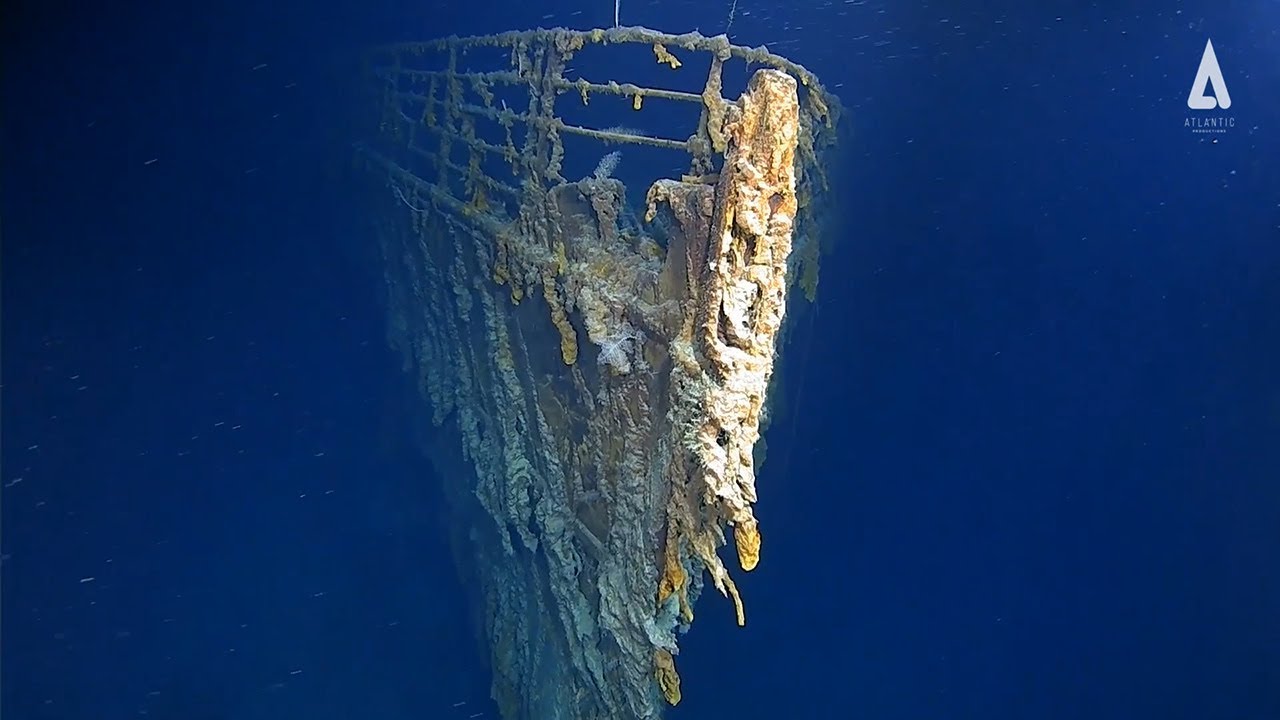The underwater photograph captures the bow of what appears to be the Titanic, immersed deep below the ocean's surface. Dominating the scene is the ship's railing, heavily encrusted with barnacles and various marine growth due to prolonged submersion. The deep, dark blue of the water underscores the great depth at which the wreck sits, with the murky hues illuminated by the camera's flash. The bow's rusting structure is enveloped in a mix of whites, dark blues, grays, tans, and yellows, presenting an eerie, yet captivating look at the decaying majesty of the once-iconic vessel. In the upper right corner of the image, an emblem labeled 'Atlantic' is visible, though smaller accompanying text remains unreadable. Scattered white dots, likely particles or small marine organisms, add to the scene's authenticity and haunting beauty.